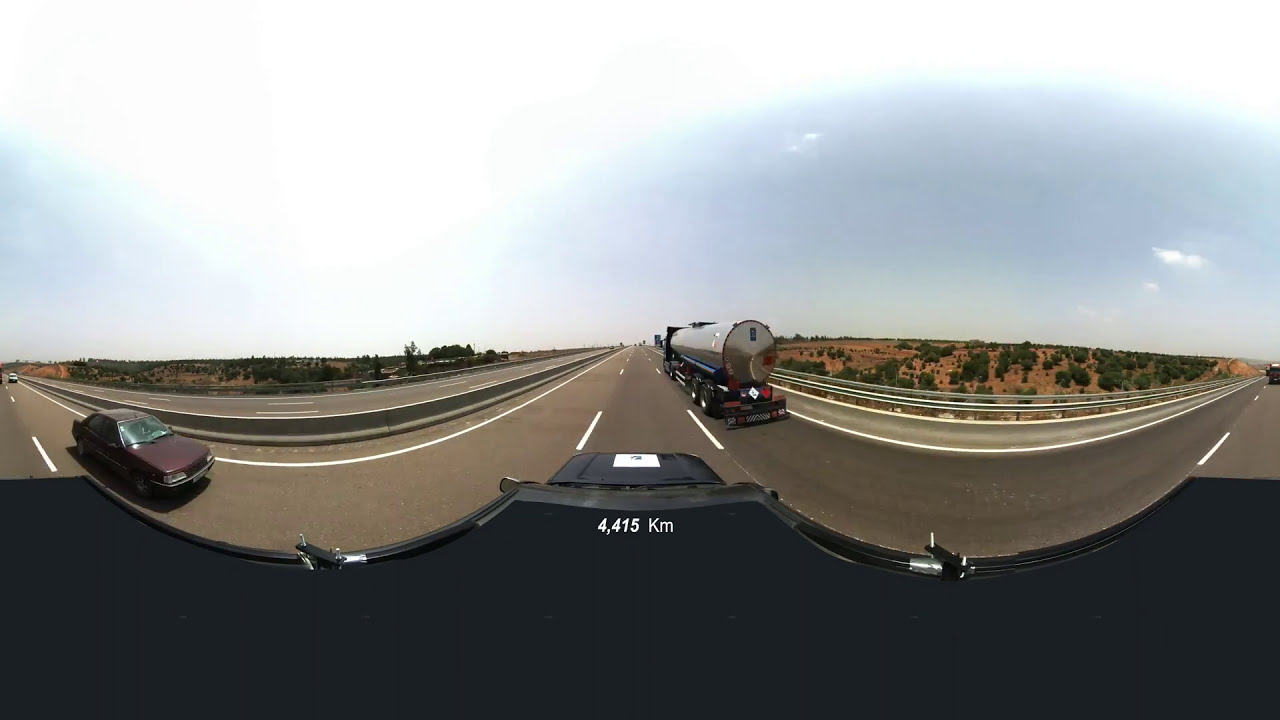This captivating photograph, taken from a vantage point atop a semi-tractor trailer, showcases a bustling three-lane highway scene. In the middle lane, where the truck is positioned, a shiny steel tanker truck, about the same height, is seen in the adjacent right lane, presumably carrying gas. To the left, a smaller black car maneuvers alongside the semi. The roads are bordered by guardrails, leading into a central lane.

The setting includes a dramatic landscape with a valley on the right, rock cliffs adorned with scattered vegetation, and a stretch of trees and dirt behind the guardrails. On the left side of the road, more trees stand scattered in the distance. Intriguingly, the image appears to have been captured with a lens that distorts the periphery, making the road appear as if it is splitting apart towards the edges, giving it an unusual, knife-cut visual effect. 

Above the scene, the sky transitions from a blue hue to a white haze, with clouds forming at the top. A faint rainbow begins to emerge from the clouds, displaying only its blue and pink edges. The combination of the unique perspective from the truck and the dynamic roadway scene, paired with the natural landscape and atmospheric elements, makes for a thoroughly engaging and detailed depiction.